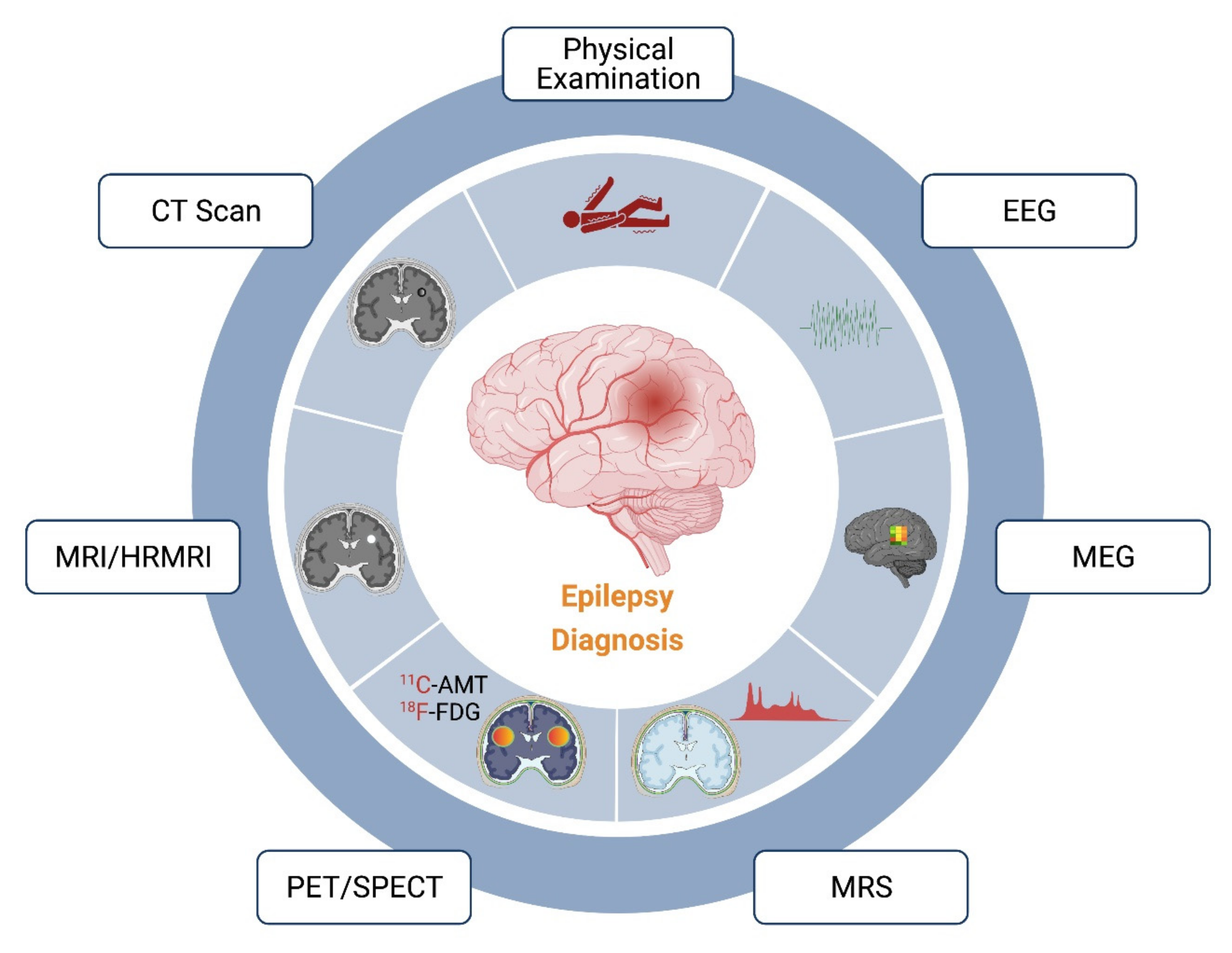This detailed medical infographic, titled "Epilepsy Diagnosis" in orange text, features a central image of a pink human brain with a red-highlighted section, all enclosed within a white circle. Surrounding this central circle is another ring divided into seven pie-shaped sections, each illustrating different diagnostic procedures. Clockwise from the top, the sections are labeled "Physical Examination" (featuring a fallen figure), "EEG" (with a brain scan reading), "MEG" (depicted by a gray brain with a colorful figure), "MRS" (with a half-brain and red graph), "PET/SPECT" (another gray half-brain), "MRI/HRMRI" (a blue half-brain), and "CT Scan" (a gray half-brain). The outermost layer of the infographic is a blue circle punctuated by white boxes that further label and highlight each diagnostic procedure.